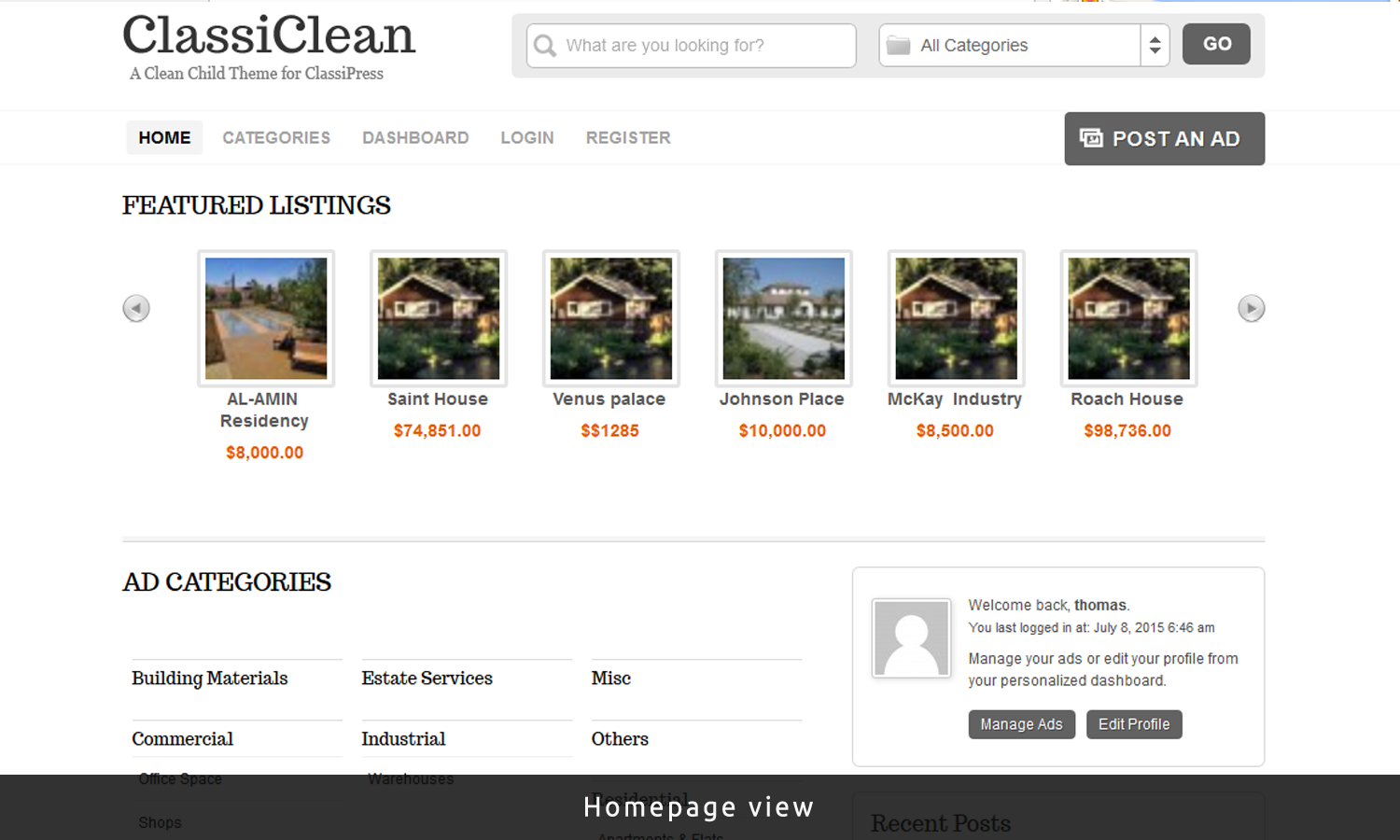This image is a detailed snapshot of a webpage for "Classy Clean," which is described as a clean child theme for Classy Press. The top section features a prominent search box with the placeholder text "What are you looking for" accompanied by a grey magnifying glass icon. Adjacent to it, there's a categories filter and a grey "Go" button.

The navigation bar includes sections labeled Home, Categories, Dashboard, Login, and Register. Below this, there's a "Featured Listings" section displaying various properties with images and details. The listings are:

1. **All-Men Residency** - depicted with an image of a setting with two lanes of water and an outdoor seating area.
2. **Saint House**
3. **Venus Palace**
4. **Johnson Place** - noted for its larger appearance compared to other properties.
5. **McKay Industry**
6. **Roped House**

Many of the listings use the same image of a small brown house. The properties vary significantly in price, starting from as low as $8,000 and going up to $74,851, with another at $1,285.

At the bottom of the page, there are additional filters under "Add Categories," listing options such as Building Materials, Estate Services, and Commercial Industry. 

The page includes a personalized message: "Welcome back, Thomas. You last logged in on July 8th, 2015, at 6:46 AM." Below this message are options to manage ads or edit the profile, with corresponding grey buttons.

The overall design of the website features a clean, predominantly white background with black text, interspersed with grey buttons for various actions.